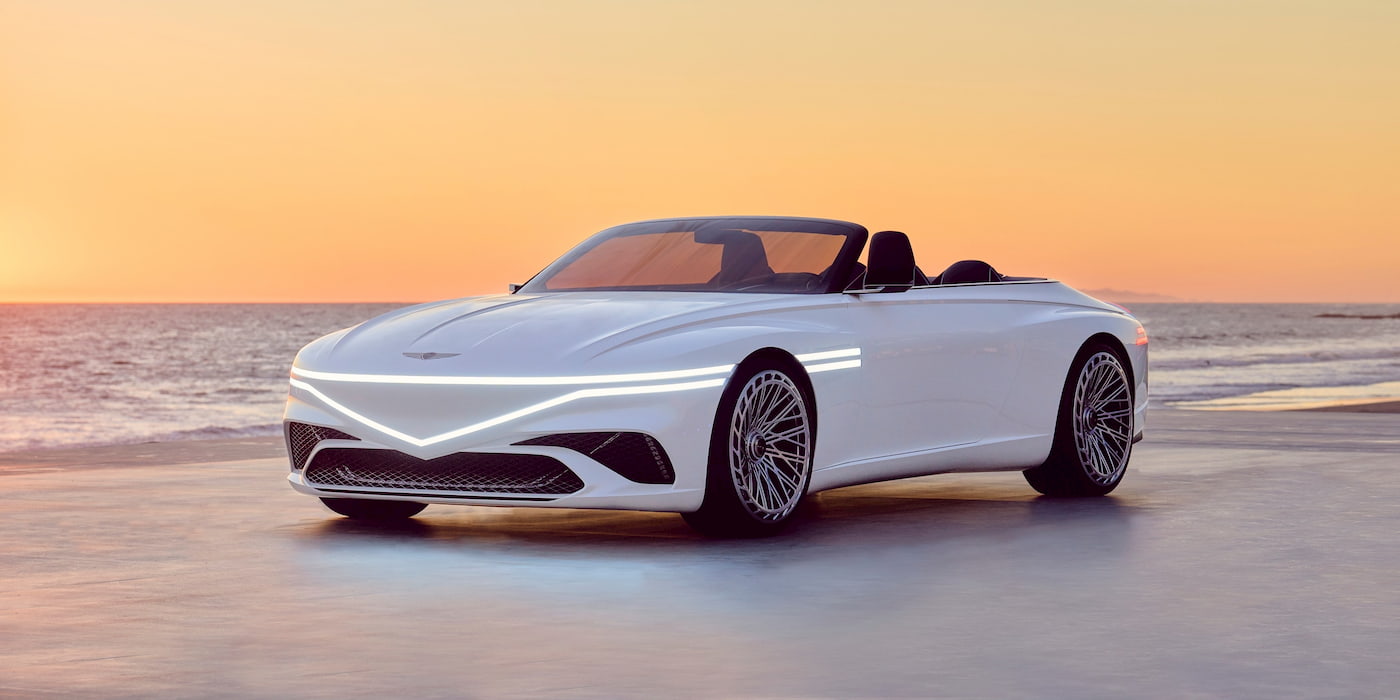The image showcases a striking scene of a sleek, white sports convertible parked on a smooth, firm sand beach against the backdrop of a stunning sunset. The sky is painted in light orange and yellow hues, blending seamlessly with the horizon where the ocean meets the sky. The car, with its top down, reveals elegant black seats and boasts a futuristic design with unique, triangle-lined LED headlights. The headlights are thin, white stripes, adding to its modern look. The sporty vehicle features seamless two doors and ornate, silver hubcaps that dominate the wheels. Its distinctive styling suggests it could be a high-end make, possibly a Bentley or a Genesis. The setting sun casts a golden glow on the sand, enhancing the overall serene beach atmosphere.